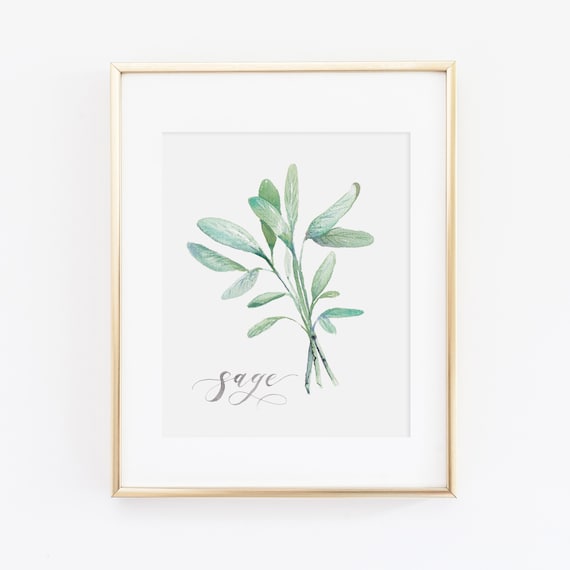This is a detailed image of a framed artwork depicting an herb. The frame features a gold trim and glossy finish, and it is mounted on a clean, white wall. Inside the frame, there is an artistically rendered watercolor drawing of a sage plant. The sage is bundled together and drawn at a diagonal, with its leaves and stems appearing in a rich olive green hue. The drawing is centered within a paper mat that has a soft gray background, mirroring the light gray tone of the overall background. Near the bottom left of the artwork, the word "sage" is elegantly written in dark gray cursive script, clearly identifying the herb. The entire piece is encased under glass, adding a refined touch to the presentation.